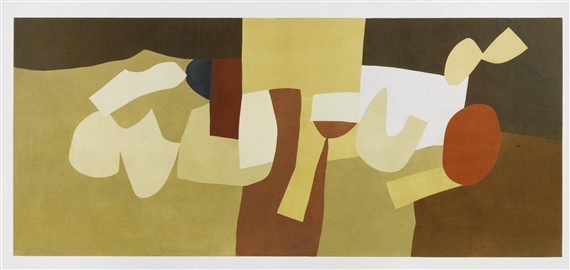The image is a detailed abstract painting featuring an array of irregular, yet distinctive shapes and patterns. Dominated by various shades of brown ranging from dark to light, the top left section showcases a dark brown area that extends to the center. Beneath this, a mustard green section appears with two beige-colored, irregular shapes—a slanted line resembling an upward stroke and a 'W'-like formation, followed by an 'L'-shaped structure. In the middle section, the upper part transitions to mustard yellow while the lower part is brown, and within this region, a white and brown cup stands out. The right section features a gradient from dark brown at the top to lighter brown at the bottom, highlighted by a prominent light brown oval shape that bridges both dark and light sections. The overall composition is a complex interplay of large, undefined shapes portrayed in earthy tones and mustard yellow, with the suggestion of a red circle and a potential interpretation of a wine glass, inviting viewers to explore and interpret the artwork individually.